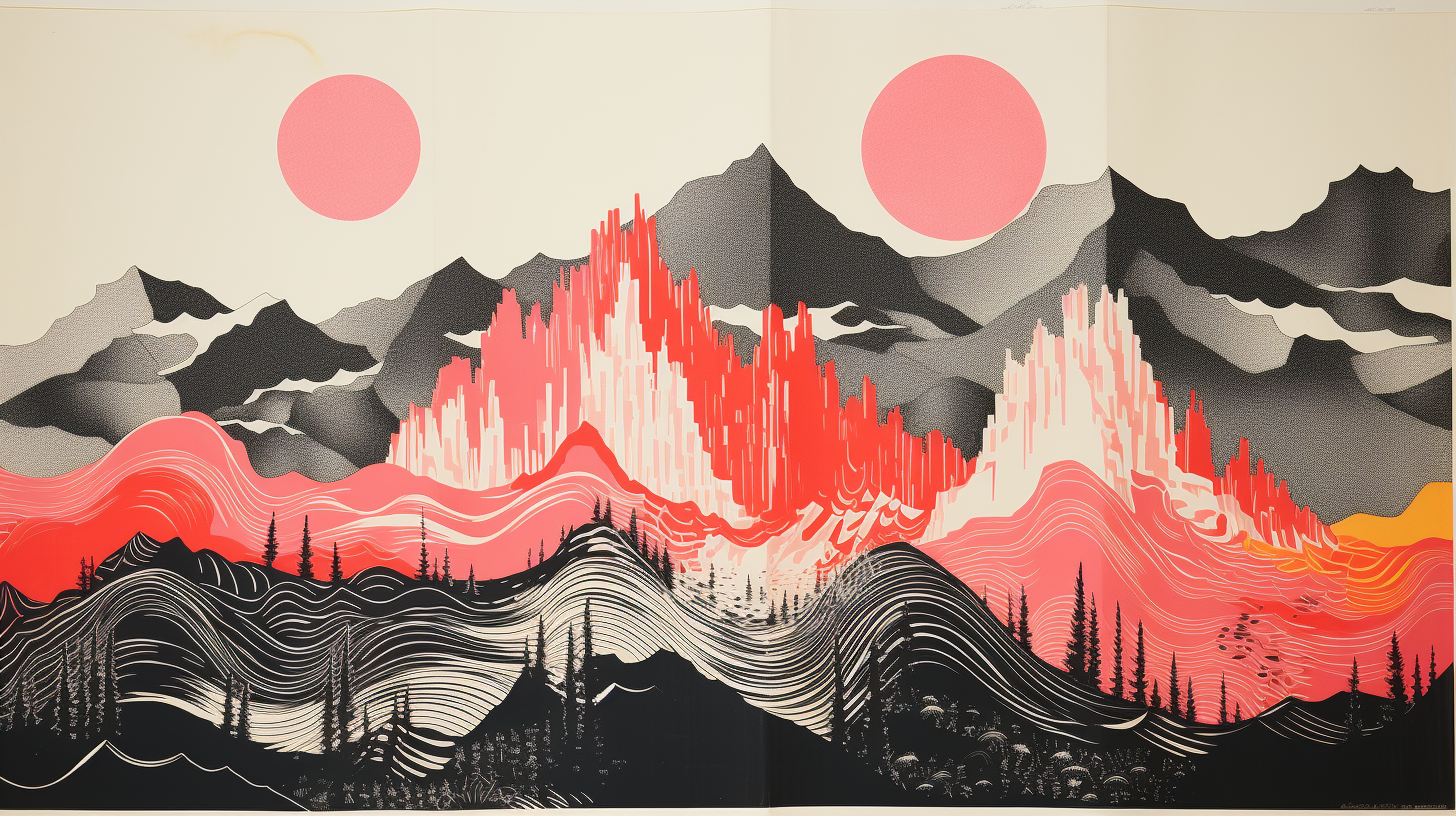This is a richly detailed illustration depicting an alien world with two pink suns set against a tan sky. The scene is an abstract creation, possibly drawn with ink or colored pencils, featuring various layers and intricate details. In the background, gray and brown mountains rise up, capped with white snow. In front of these mountains are more jagged, pointy peaks colored in shades of pink, red, and white, resembling ice. Two rivers flow at the base of the mountains: one in hues of pink and red, and another in black and white, giving the impression of swirling, dynamic movement. Pine trees silhouetted against the landscape add a touch of familiar earthiness to this otherworldly scene. The entire image evokes a sense of a futuristic or fantastical planet, blending natural elements with imaginative, striking colors.